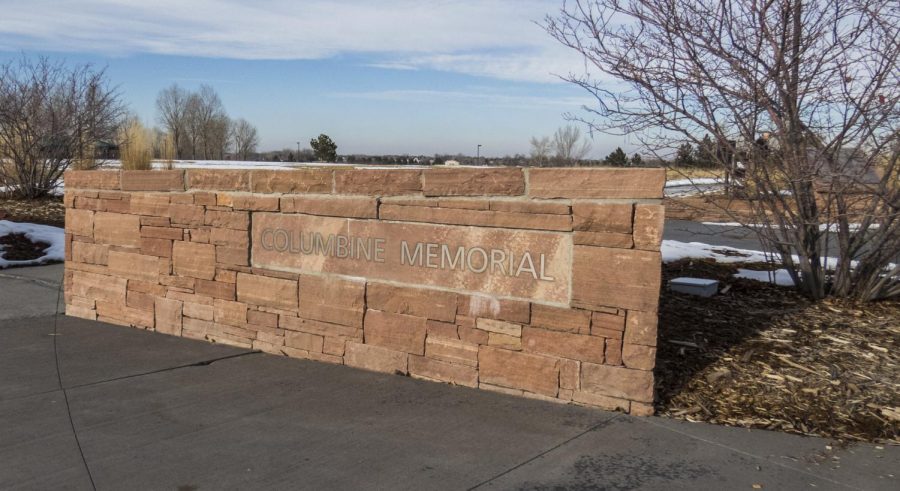The color photograph captures a meticulously built Columbine Memorial stone wall, approximately 15 feet long and 4 feet high, situated at the edge of a sidewalk. The wall, constructed from an array of square and oblong beige and cream-colored stones set in a random pattern, features a prominent horizontal rectangular plaque near its top, inscribed with "Columbine Memorial" in white text. The surroundings include several flower beds and a partially snow-covered parking lot, contributing to the cold, wintry atmosphere. Barren trees and hay patches in the background, along with a narrow pond, suggest a somber scene. The bright sky overhead enhances the stark, reflective quality of the memorial site. The image is in landscape orientation and conveys a sense of photographic realism, capturing the texture and details of the wall and its surroundings with clarity.